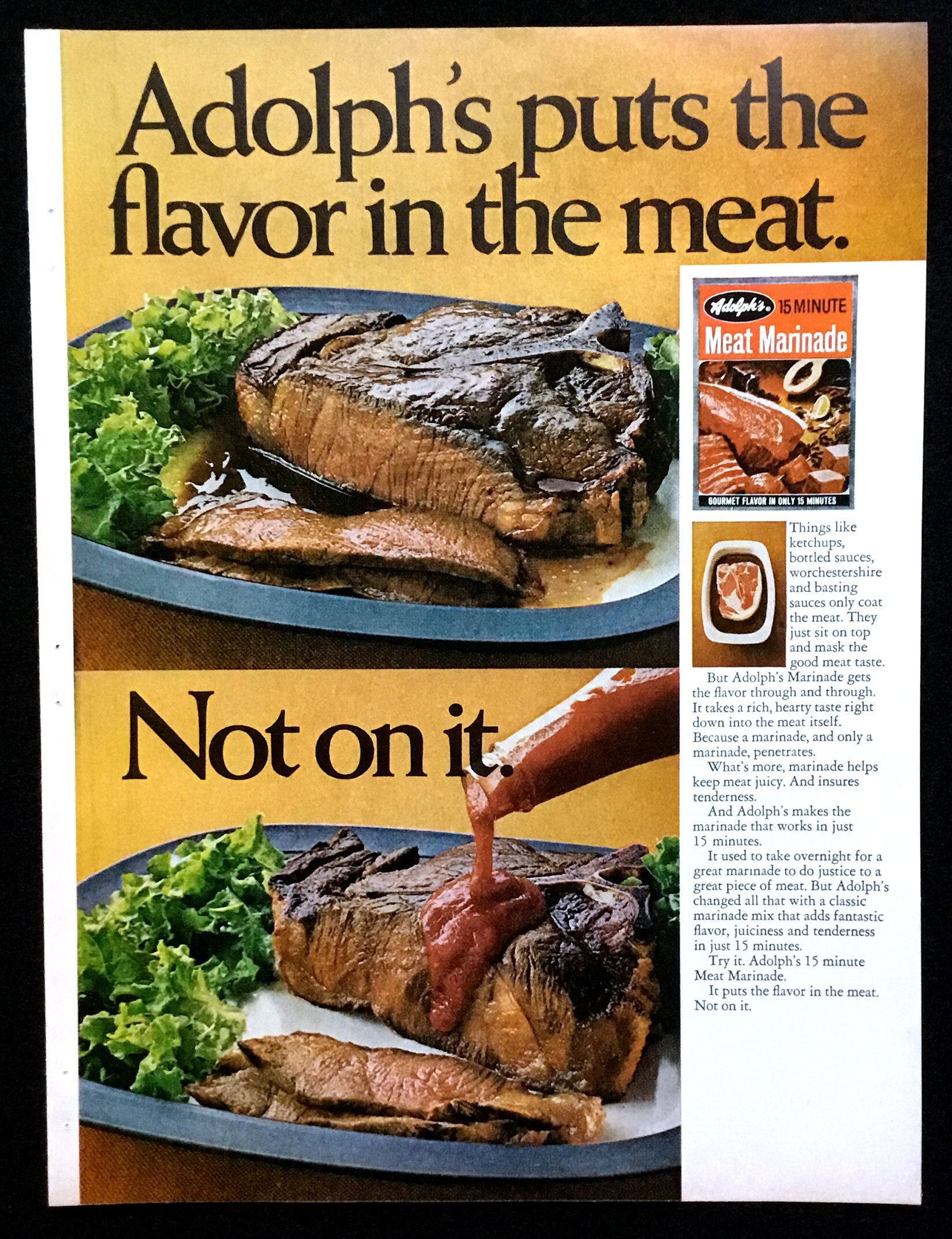The image appears to be a page from a magazine or an advertisement for Adolf's 15-Minute Meat Marinade. The main body of the page prominently features two images of steak on blue and white plates garnished with green leaves. The top image displays a large New York steak cut into long strips without any sauce, emphasizing Adolf's slogan, "Adolf's puts the flavor in the meat." The bottom image shows a similar steak with red sauce poured over it from a clear bottle, accompanied by the text "not on it." To the right, there is a detailed instruction box for the marinade, showcasing the packaging of Adolf's 15-Minute Meat Marinade. The packet, set against an orange background, features an image of a marinated steak and outlines the proper usage of the marinade.